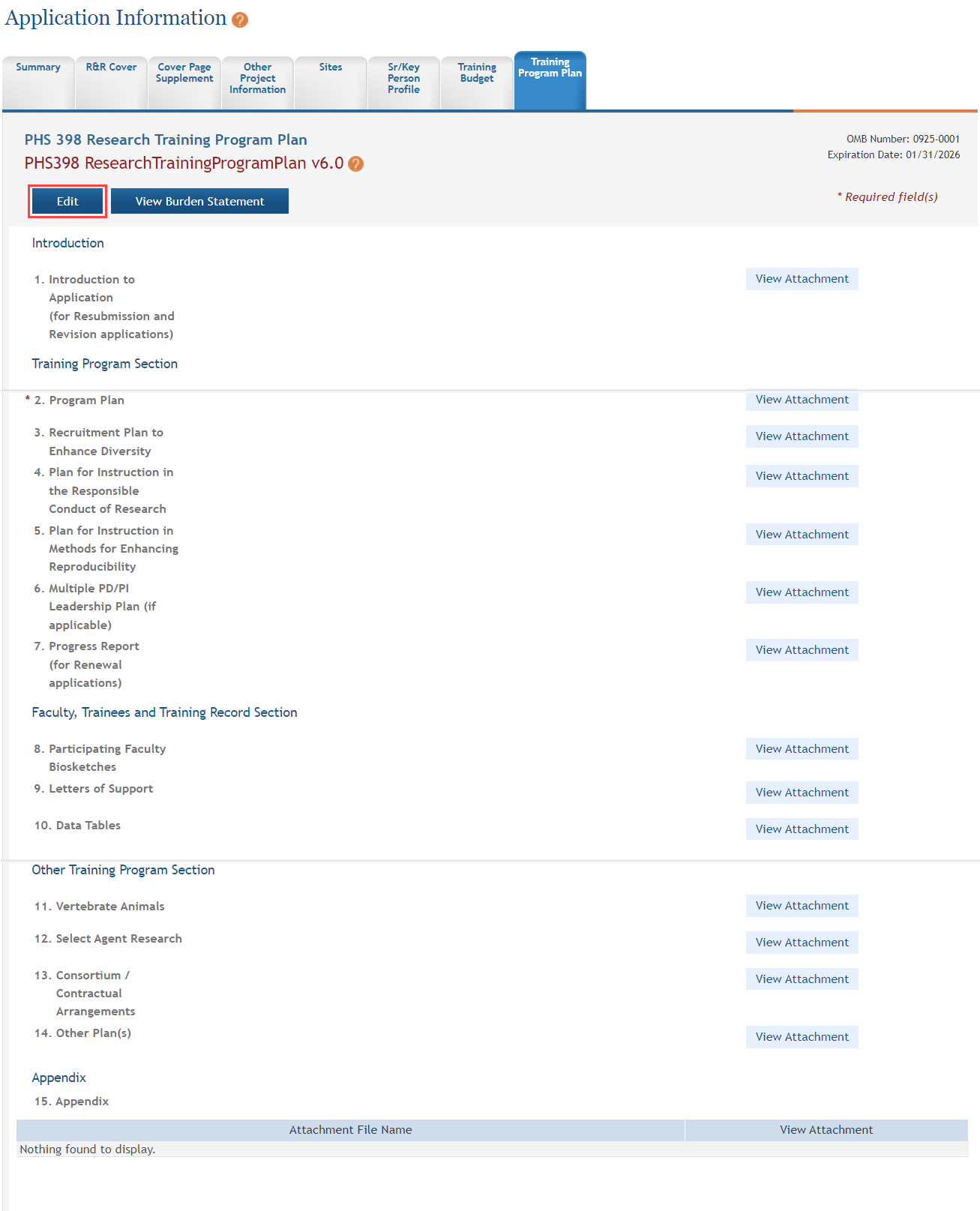Screenshot of a website displaying application information at the top in blue font on a white background. Below the header is a horizontal menu consisting of gray tabs with blue text, listing options such as Summary, R&R Cover, Cover Page Supplement, Other Project Information, Sites, SR/Key, Person Profile, Training Budget, and Training Program Plan. The Training Program Plan tab is highlighted in blue, indicating it is the selected section.

Underneath the menu is a gray rectangle with blue text that reads "PHS 398 Research Training Program Plan." Just below this, in red text, it states "PHS 398 Research Training Program Plan Version 5.0." On the right side of this gray rectangle is the OMB number "0925-0001" and the expiration date "10-31-2025."

The main content area below the gray rectangle features a white page with blue text, starting with the heading "Introduction," followed by "Introduction to Application for Resubmission and Revision of Applications."